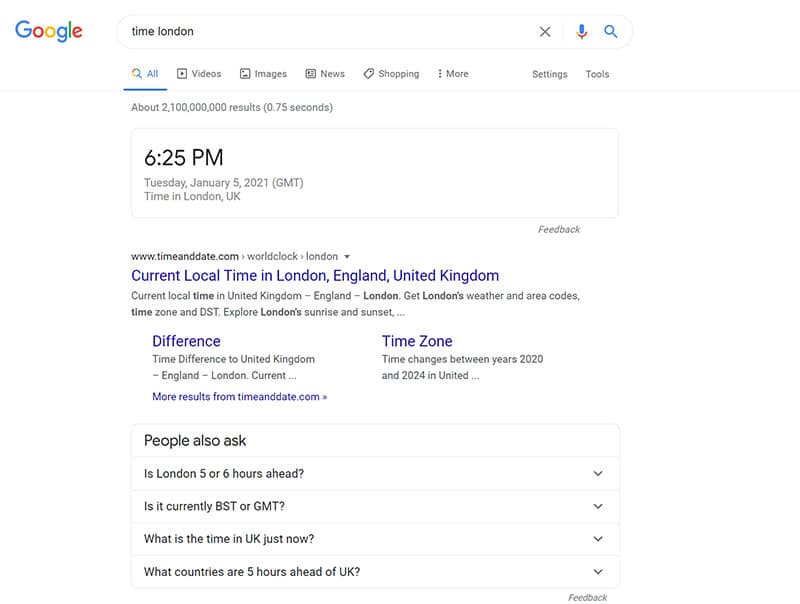Sure, here's a cleaned-up and detailed caption:

---

The image displays a Google search results page. In the top left corner, the iconic Google logo is prominently featured. Below the logo is an elongated search bar containing the query "Time London." To the right of the search bar is an 'X' icon, followed by a vertical line that separates it from a microphone icon and a blue magnifying glass icon.

Directly beneath the search bar is a secondary horizontal menu bar. This bar includes various search categories, each represented by corresponding icons and text labels. From left to right, these categories are: "All" (highlighted with a blue underline), "Videos" accompanied by a box with a right-pointing arrow, "Images" next to an image icon, "News" paired with a news icon, and "Shopping" which is indicated by a shopping tag icon. Next, there are three vertically stacked dots encompassing the "More" options, followed by "Settings" and "Tools."

Proceeding down the page, a text line reveals that there are about "2,100,000,000 results (0.75 seconds)" for the search query. Below this line is a gray rectangular box with a thin white border. Inside this box, it states the current time as "6:25 PM, Tuesday, January 5th, 2021 (GMT)" along with the text "Time in London, UK." In the lower right corner of the box, there is a "Feedback" link.

Finally, the page begins displaying the list of search results starting with the first website.

---